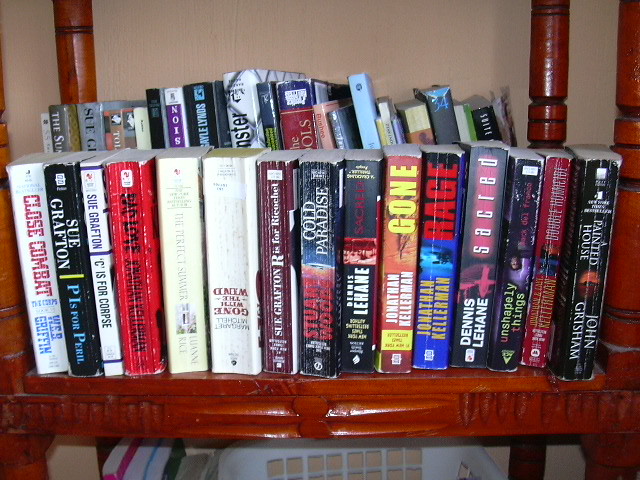This color snapshot photograph captures a close-up view of two rows of paperback and hardcover books arranged on the lower shelf of a reddish mahogany-colored wooden table. The front row consists of medium-height, vertically standing paperback books, some of which are upside down, displaying clear signs of wear. Notable titles in this row include "Close Combat" by West Griffin, "Cold Paradise," "Gone," "Rage," and "Phantom House" by John Grisham. The back row comprises a mix of taller paperback and hardcover books and is slightly blurred, indicating it is positioned further back. Both rows are photographed against a light brown wall. The wooden table features dual levels, functioning as a small bookshelf on the lower one. At the bottom edge of the photograph, a white laundry basket is visible. The image appears to have been taken with a flash, illuminating the scene and highlighting the wear on the books and the wood grain of the shelf.